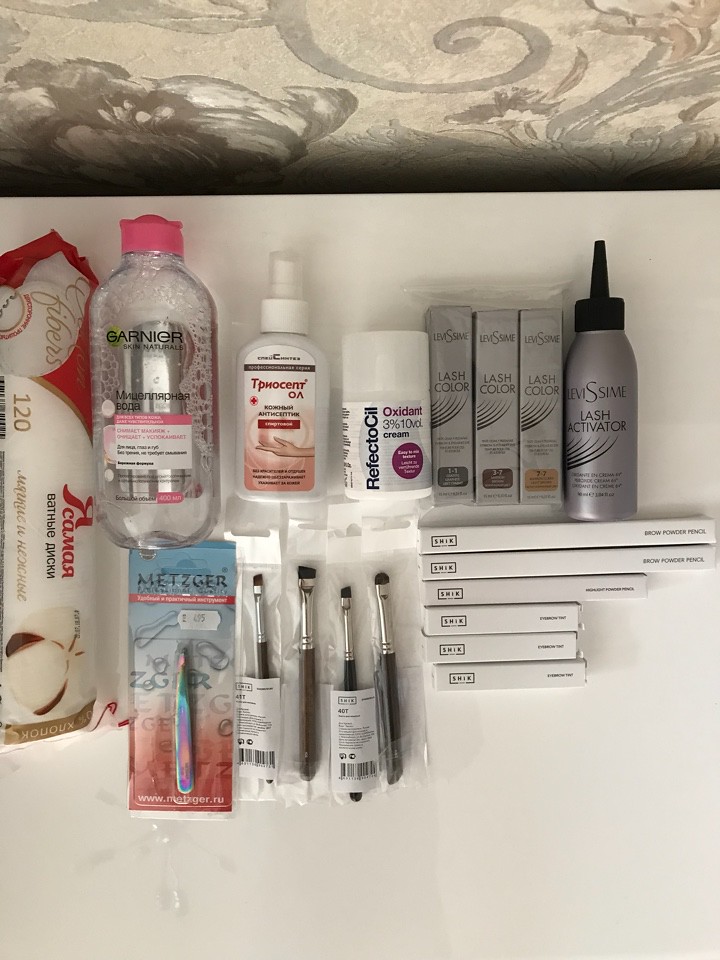This image showcases a meticulously arranged assortment of beauty products on a white table, viewed from an overhead perspective. At the top edge of the image, there is a taupe-colored background, possibly the back of a couch or wallpaper, featuring a delicate flowery design with swirling stems in darker and lighter shades. A black shadow creates a distinct separation between this flowery backdrop and the white table holding the beauty items.

From left to right, the first item appears to be a package of cotton rounds labeled with the number 120 in a language resembling Russian. Next to it is a Garnier bottle containing a liquid with bubbles, distinguishable by its pink cap. Adjacent to the Garnier bottle is a smaller white spray bottle featuring text in a foreign language and displaying a Caucasian hand pointing leftward.

The following item is a Reflectocil oxidant cream, marked with "3% 10 volume" and a purple circle with white text that is too small to read clearly. To its right are three narrow gray boxes by Le Sam, labeled "Lash Color" with illustrated eyelashes below the text. Each box displays a different colored small square at the bottom: gray, brownish, and tan, respectively. These boxes are neatly placed together in a single plastic container.

To the left of these boxes, there is a product labeled Lash Activator, beneath which several white boxes of varying sizes are visible. On the lower level, moving leftward, we see an array of makeup brushes. The rightmost brush has a domed head, followed by three slanted brushes of varying sizes; the slant directions alternate between right and left. Finally, there is a package of tweezers by Metzger, featuring pastel-colored tweezers.

This organized ensemble of beauty products reflects both diversity and meticulous arrangement, creating an inviting and well-ordered visual presentation.